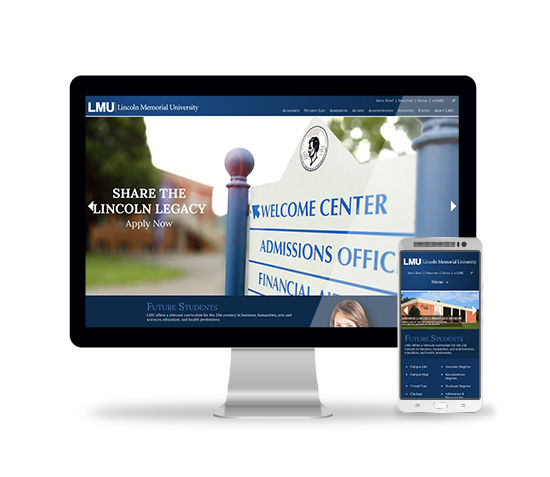The image features a white computer with a black-rimmed screen displaying a webpage from Lincoln Memorial University (LMU). At the top of the screen, a blue banner showcases the LMU logo with the text "Lincoln Memorial University" in small white print and a white 'X' in the corner. Below this, a photograph of the University greets visitors with a sign that reads "Welcome Center, Admissions Office, and Financial Aid." 

In the center, there is a promotional message: "Share the Lincoln Legacy - Apply Now," accompanied by a left arrow pointing towards options for future students. The lower part of the screen also highlights future students’ resources against a darker blue background. The top of a person’s head is partially visible near this section.

On the right side of the screen, there is an image of a white telephone beside another LMU logo set against a dark blue background. A picture of a picturesque brick University building with a white top is featured, along with navigational white arrows pointing left and right. The bottom section of the screen is predominantly white, possibly containing additional information or links.